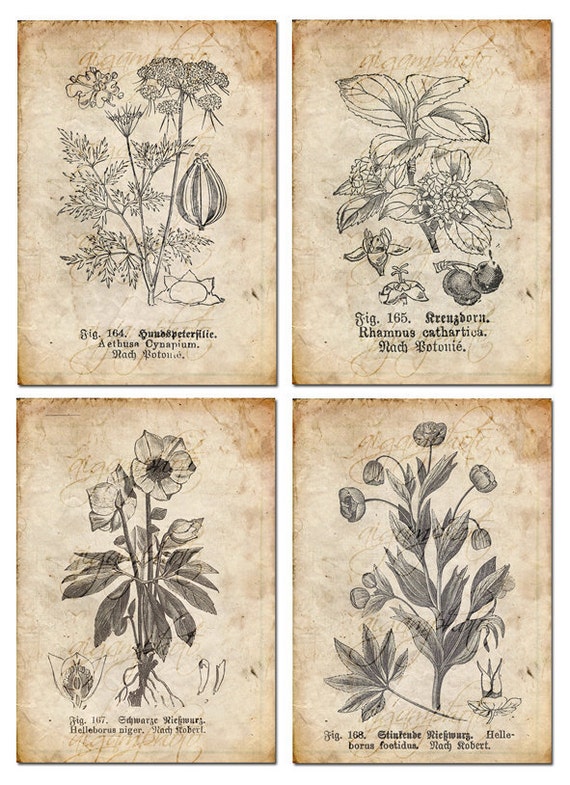The image features four separate botanical illustrations on old, parchment-style pages arranged in a 2x2 grid against a clear white background, with white lines separating each page. The paper appears tea-stained, darker around the edges, and lighter in the center. The illustrations are highly detailed pencil sketches, predominantly in black or gray, showcasing various plants, most with flowers. Each drawing is accompanied by a caption in black text providing the plant's figure number and scientific name. The upper left image, labeled "SIG 164," depicts a flowering plant with an intricate, albeit partially unclear scientific name. The upper right illustration, numbered 165, shows Gremsborn Ramnus cathartica rot botany. In the lower left, figure 167 is a detailed drawing of Helleborus niger. The lower right corner features figure 168, labeled as Stentend riffurg, Helleborus foetidum, with delicate bell-shaped flowers. These pages appear to be from a historical botanical book, capturing the delicate artistry and scientific labeling of plant specimens.